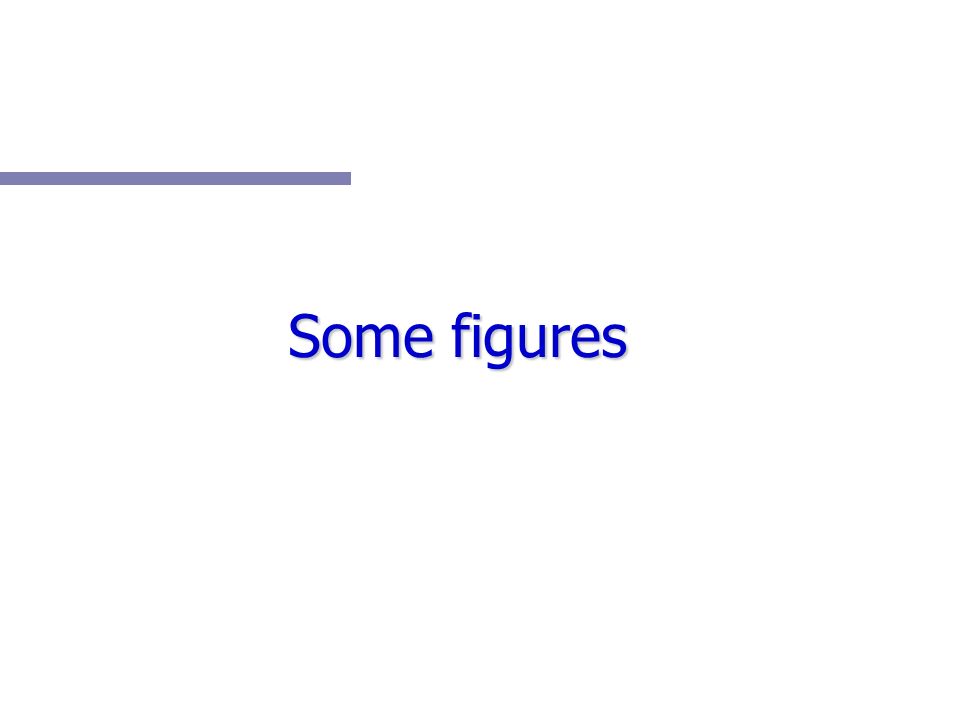The image features a pristine white background. In the top left corner, there is a thick, horizontal bar extending halfway across the image. This bar, described variably as a medium-shaded blue or a steel gray with a hint of purple, carries a distinctive subdued tone. Below this bar, centered in the image, are the words "SUM FIGURES" in a bold, vivid navy-blue, sans-serif font. The capital "S" in "SUM" contrasts with the lowercase "f" in "FIGURES". The text stands out more brilliantly against the white background than the horizontal bar does, creating a striking visual focal point. There is approximately an inch of spacing between the bar and the text, making the elements distinct yet related. The simplicity of the image and the choice of colors evoke a clean and modern aesthetic.